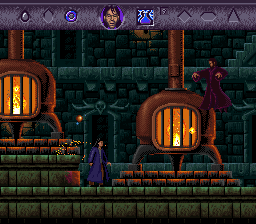A detailed screenshot from a mobile or computer video game features a square graphic with meticulously designed green stone steps and gray stones forming the background. Dominating the scene are two wood-burning stoves, one prominently raised towards the left and the other just right of the center. These stoves, cast in a warm brownish-bronze hue, emit a lively orange glow from the fires crackling within, with slender chimneys stretching upwards from each. Floating above the right-hand stove is a man draped in a dark burgundy robe, peering downwards with intent, seemingly towards another character. This second figure, positioned to the left of the same stove, is adorned in a deep blue robe that emits a cascade of sparkles. Crowning the image at the very top, a gray bar stretches horizontally, featuring a small portrait of a person alongside a quaint graphic of a potion bottle.